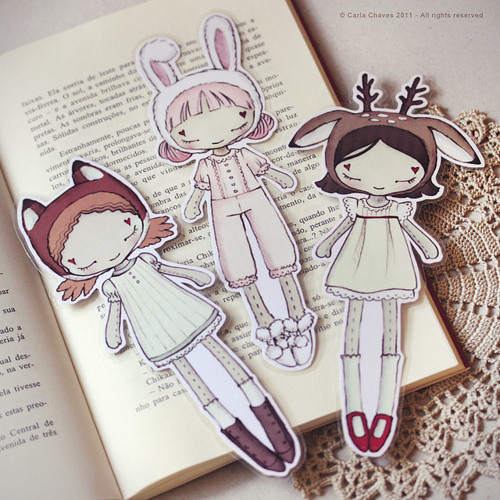The image features three cartoonish paper dolls or bookmarks laid flat on the right page of an open book, which is diagonally oriented at approximately a 40-degree angle to the left. The book has printed black text on white pages and rests on a table covered with a lace doily.

Each doll character has distinct features and attire, yet they share the common detail of having their eyes closed with purple hearts above them. The first character on the left has red hair, a white dress, white socks, and brown boots, topped with a beanie-like hat featuring cat ears. The middle character sports pink hair and a white-and-pink bunny hat. This character is dressed in a short-sleeve blouse and knee-length pants, completed with white slippers. The character on the right has dark brown hair, a reindeer hat, a beige short dress, white knee socks, and red buckle shoes.

The upper right corner of the image contains the text "Carla Chaves, 2011, All Rights Reserved."